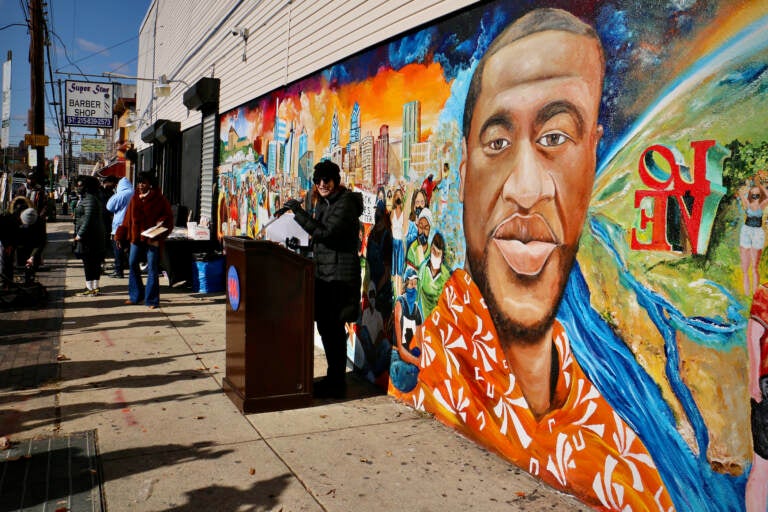In this outdoor photo, a detailed mural adorns the side of a building, featuring a powerful depiction of George Floyd, an African American man famously murdered by a police officer in Minnesota. The mural reveals Floyd dressed in an orange and white Hawaiian shirt, his visage strikingly fixed on the wall amidst a colorful rainbow-influenced background. The word "LOVE" is prominently displayed on this vibrant artwork. 

A woman, clad in all-black attire including a hat and sunglasses, stands at a brown wooden podium bearing a circular emblem, positioned at a 45-degree angle. She appears to be addressing an audience to her left. Behind her, the mural extends to include various elements: graffiti-like portrayals of city skylines, pedestrians, and earth-like imagery. The left side of the mural notably features a sign reading "Superstar Barbershop." The scene includes noticeable details such as a concrete sidewalk lined with people and telephone poles, reinforcing the urban setting. The sky in the background shows a deep blue with minor clouds, adding a serene contrast to the compelling subject matter.